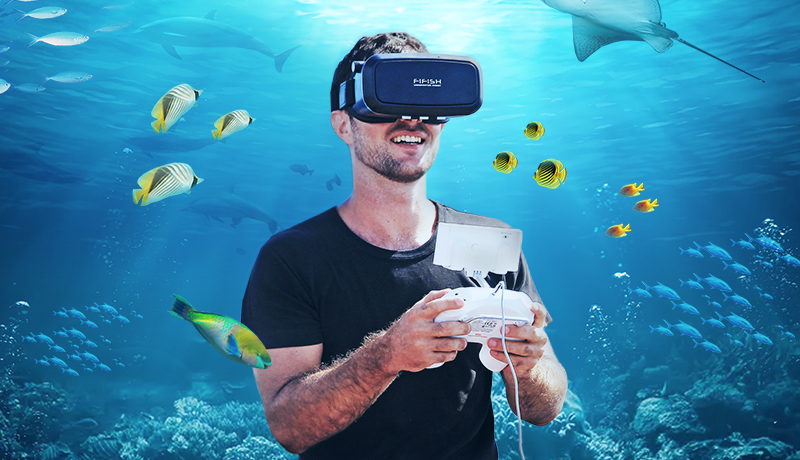The image depicts a man immersed in a virtual reality experience. He is wearing a large VR headset, which has an attached wired controller that he holds in one hand. The controller appears to have a smartphone set in it, further tethered by a cable. He is dressed in a black t-shirt, and has short dark hair, a stubble beard, and a tattoo on his arm. The backdrop of his virtual world features a vivid underwater scene, complete with crystal blue water and a variety of marine life, including yellow, black, and white fish, stingrays, a shark, dolphins, and possibly a whale. The man has a pleasant expression on his face, suggesting he is enjoying the virtual dive into this aquatic environment.